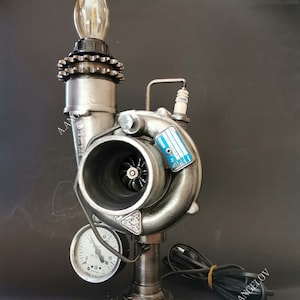The image showcases a detailed and intriguing steampunk-inspired sculpture created from various found metal parts. At its core, the sculpture features a central, fan-like component resembling a meat grinder or turbine, meticulously fashioned from dark gray aluminum. This central structure is intriguingly tubular, reminiscent of a tuba, and is accented with two gleaming silver gears at the top.

On the lower left side of the sculpture, there is a circular pressure gauge with a black meter. This gauge appears to monitor or add an element of functionality to the piece. Rising from the upper left, an old-fashioned candelabra-shaped bulb is mounted in a brown plastic socket, formerly bakelite, attached to the main structure via a bent piece of metal. The exposed internal elements suggest a visually compelling deconstruction of machinery.

Notably, a spark plug is visible, suspended amid the assembly, adding to its intricate, mechanical aesthetic. The entire contraption, which suggests a lamp-making kit, is secured with a wound brown electrical cord, tied neatly with a twist tie or rubber band.

The sculpture also bears a watermark with the name "Angelove", indicating the creator’s signature. This well-crafted piece stands as an imaginative fusion of metal, technology, and art, illuminating the whimsical and industrial steampunk genre.